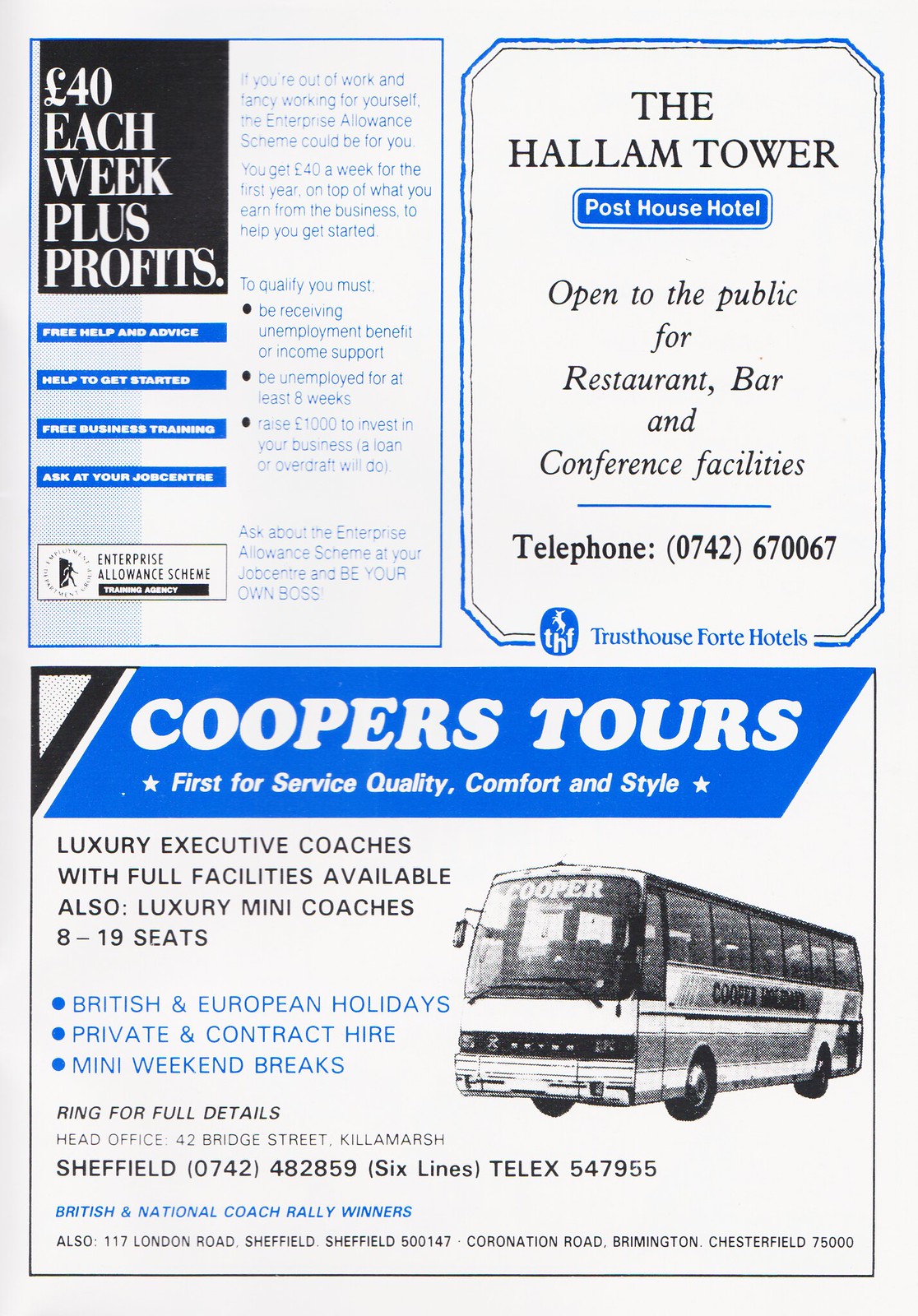The image depicts a detailed advertisement page from a magazine or newspaper, featuring three distinct ads set against a predominantly white background with black and blue text. The upper half of the page is divided into two ads: 

1. On the left, an ad for the "Enterprise Allowance Scheme" is set against a black background with white letters stating, "£40 each week plus profits." The ad provides additional information in blue text, promoting free help and advice, business training, and the opportunity for self-employment through the scheme. It suggests asking at the job center for more details.

2. On the right, an ad for the "Hallam Tower Post House Hotel" invites the public to enjoy its restaurant, bar, and conference facilities. The ad, titled in black letters, promises quality service and includes a telephone number for reservations. It's part of the Trust House Fort Hotels chain.

The lower half of the page features a single ad:

3. This ad promotes "Cooper's Tours," highlighting its first-rate service, quality, comfort, and style. The ad, set against a blue background with white letters, includes a black-and-white illustration of a bus labeled "Cooper." It provides detailed descriptions of the luxury executive coaches' facilities, along with contact information including telephone numbers and addresses.

The overall design is well-organized, ensuring clear visibility and easy navigation through the different ads, with a harmonious use of colors and imagery.